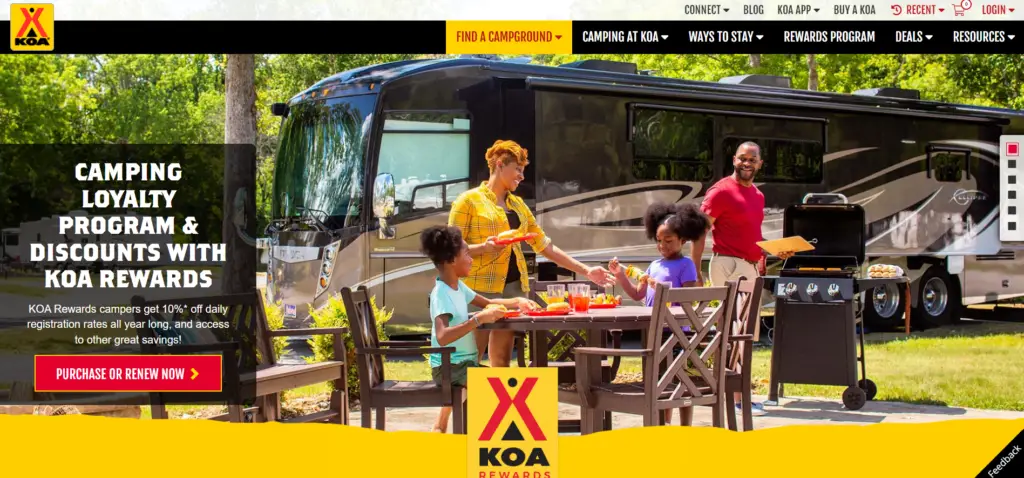This image is a detailed screenshot of the KOA Campground website in desktop format, specifically showcasing the homepage. Dominating the visual is a large RV set against the backdrop of an African-American family enjoying an outdoor meal with table and chairs, depicting a quintessential camping experience. The family appears to be engaged in grilling and dining activities. The focal point of the page is information about the Camping Loyalty Program, which highlights the benefits of KOA Rewards. It encourages users to register to receive a 10% discount on registration rates and additional savings. At the bottom of the page, the KOA logo is prominently displayed with the word "Rewards" underneath, reinforcing the emphasis on the loyalty program. At the top of the page, there is a navigation menu with options such as Connect, Blog, KOA App, Buy a KOA, Cart, and Login. Beneath this, a horizontally presented menu features categories like Find a Campground—which is highlighted in yellow—Camping at KOA, Ways to Stay, Rewards Programs, Deals, and Resources.